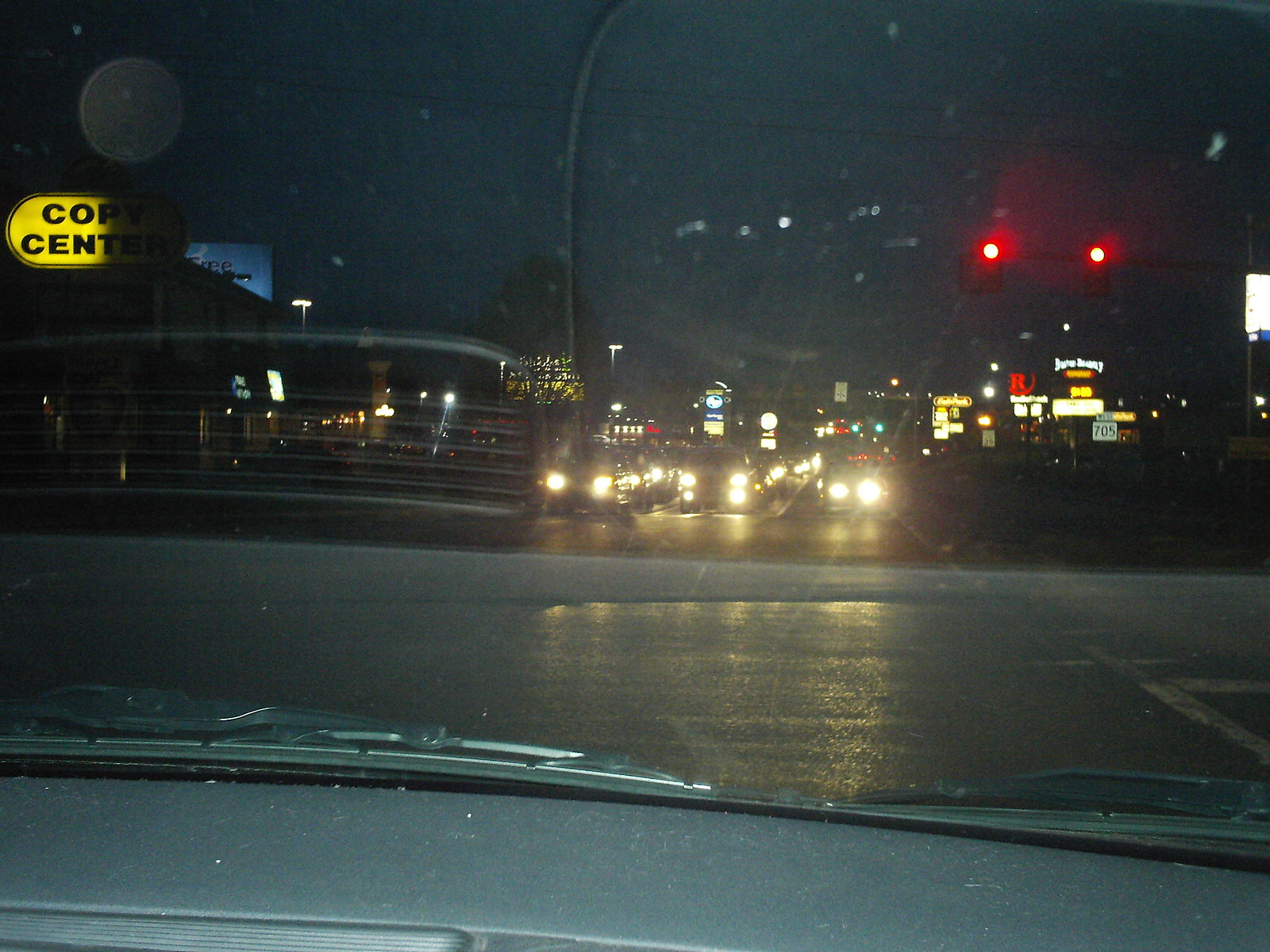This captivating color photograph captures a nighttime scene viewed through the window of a car, possibly the front or side window. The bottom portion of the image displays a faint, greyish interior of the car, setting the context for the viewer's perspective. The road ahead is enveloped in darkness, sporadically lit by scattered streetlights and the headlights of several oncoming vehicles. These cars, positioned at the central part of the image, emit bright beams that pierce through the night.

On the left side of the photograph, a section of a bridge railing adds structural depth to the scene. Meanwhile, the right side is plunged into blackness, devoid of any discernible details. In the same left vicinity, several round lights and a partially visible building emerge. This building is adorned with red, yellow, and white lights, adding a hint of urban vibrancy to the otherwise dim scene. 

In the upper left corner, a small illuminated yellow sign with black text catches the eye. The sign reads "C-O" followed by "C-E-N," possibly indicating a "Copy Center." This sign provides an additional layer of context, hinting at a commercial or urban environment.

The juxtaposition of the darkened road, the glowing lights, and the obscure car interior create a moody, atmospheric snapshot of nocturnal travel.